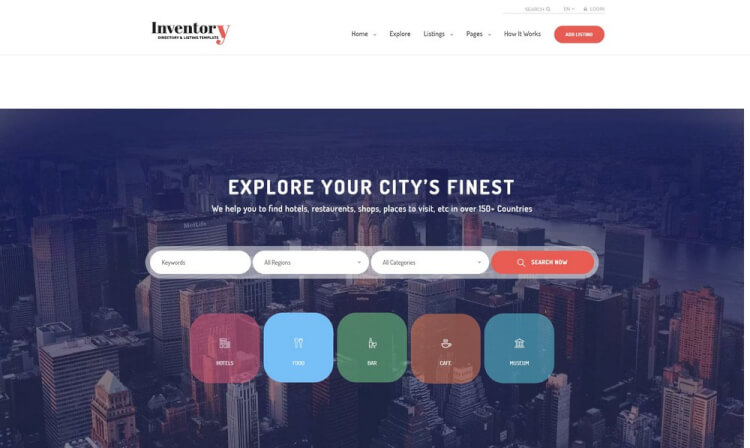The webpage titled "Inventory" appears on the top left-hand side with the word "Inventory" prominently displayed, where the 'Y' character is colored in red. Below this title, there's some blurred text that might be a description or subtitle. The webpage seems to function as a listing directory or template for various city locations. 

At the top, users can find a sign-in button, a login button, and a dropdown menu to set the language—all of which are slightly out of focus. The main menu features a series of options: "Home" with a dropdown menu, "Explore," "Listings" with a dropdown menu, "Pages" with a dropdown menu, and "How it Works." Additionally, there is a red button with white text labeled "Add Listing."

A gray bar stretches horizontally across the page from left to right, followed by a section of white space. Below the white space, a large rectangle showcases a cityscape filled with towering buildings in shades of blue, brown, and gray, along with a body of water, suggesting a vibrant metropolitan area. Overlaying the cityscape image is a white, uppercase text that reads "EXPLORE YOUR CITY'S FINEST." In smaller, lowercase white text, it further explains, "We help you to find hotels, restaurants, shops, places to visit, etc., in over 150 countries."

In the search section, users can see text boxes labeled "Keywords," "All Regions," "All Categories," and a "Search Now" button featuring a magnifying glass icon with white text.

Below this, five colored boxes represent different categories: 
1. A red box for "Hotels" with a hotel icon.
2. A blue box for "Food" with a fork and spoon icon.
3. A green box for "Bars" displaying a bottle and glass icon.
4. A brown box for "Cafes" with a steaming coffee cup icon.
5. A blue-gray box for "Museums" featuring a white museum icon and the word "Museum."

This well-structured page is clearly designed to aid users in exploring and locating various amenities within a city.